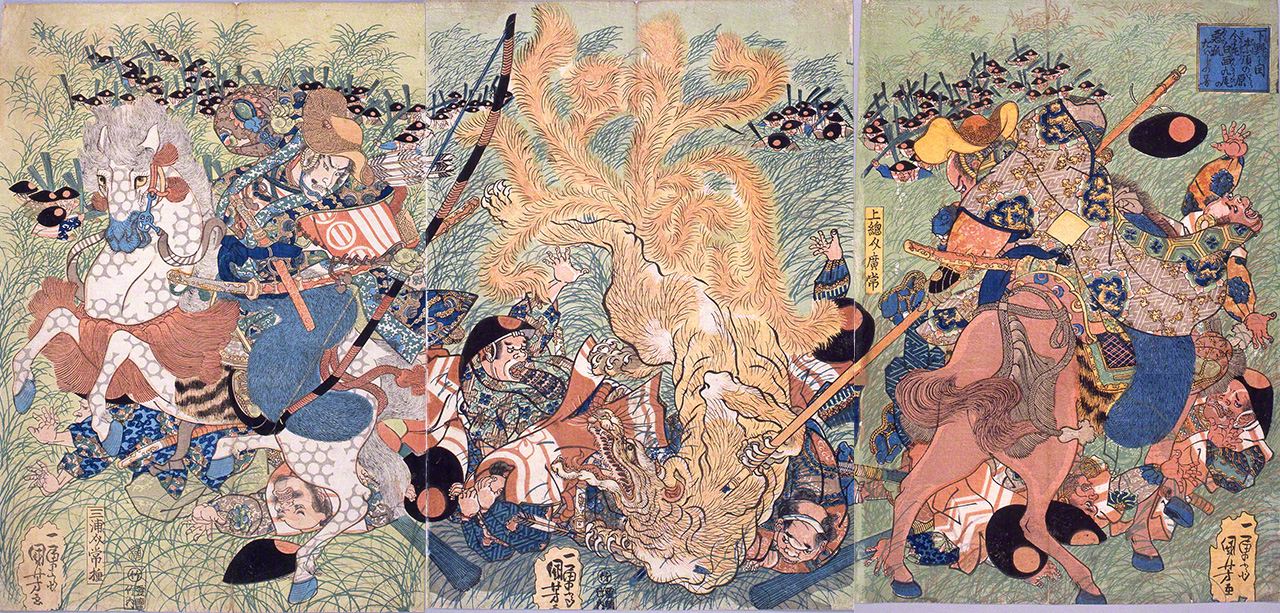This painting, rendered in an abstract style reminiscent of Picasso's Guernica, illustrates a chaotic battle scene featuring Oriental warriors on horseback, possibly from the 15th or 16th centuries. The artwork unfolds across three panels that combine to form a larger, dynamic image. The color palette prominently features various shades of brown and dark to medium blue.

In the left panel, a samurai figure in a colorful multihued armor and a flat yellow hat rides a white horse rearing on its hind legs. He holds a longbow, aiming amidst the turmoil. Soldiers trail off from the foreground on the left, moving towards the right and then downwards in a chaotic line, depicting the frenetic action of battle.

The central panel is dominated by a striking orange dragon with nine flowing tails. The dragon is engaged in combat with several warriors, some of whom are trying to restrain it. One warrior on a red horse wields a spear against the dragon. This red horse, oriented to the right and away from the viewer, contrasts with the rider who faces left, dressed in colorful garments including a robe and cloak. The dragon, with a small arm grasping one of the spears, is menacing yet vividly detailed, adding a fantastical element to the scene.

In the background, the grassy green landscape is dotted with distant soldiers holding up swords, contributing to the depth and the sense of an ongoing, larger conflict. The overall composition, with soldiers in traditional Oriental attire battling both each other and the mythical creature, creates a vivid and tumultuous narrative, teeming with movement and energy.